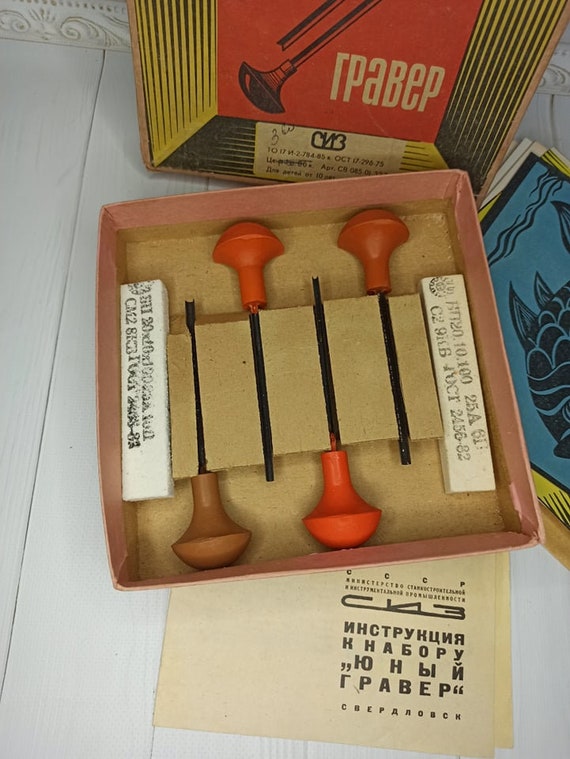This indoor photograph features a central open cardboard box displaying a set of vintage Soviet-era tools, likely chisels. The tools have handles in varying shades of orange, red, and brown, and are accompanied by black metal blades. The box's cover, situated in the background, showcases a detailed drawing of the tools in black against a vivid red backdrop, adorned with white Russian text. Additionally, the box is nestled on an underlying white, aged-looking paper with more Russian writing, indicating the set's antique nature. The scene is set on a white wooden table or floor, with white blocks of styrofoam positioned on either side of the tools, adding to the overall display.